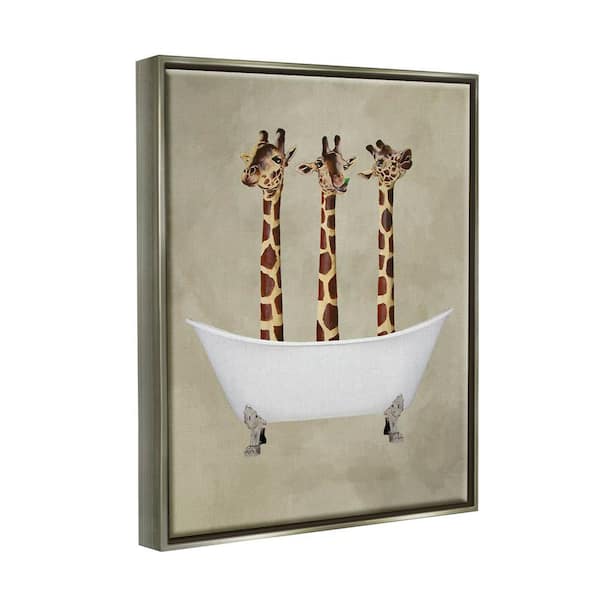The framed artwork features a quirky scene with a grayish-beige to tan-gray background, positioned at an angle where the left side is more forward than the right. It depicts three giraffe heads and their elongated necks emerging from a pristine white clawfoot bathtub, which is embellished with elegant gray or silverish claw feet. The tub is whimsically supported by two small, gray, baby cupid statues. Among the giraffes, the middle one faces forward with a green leaf in its mouth, while the giraffes on either side turn their heads in opposite directions – one gazing to the left and the other tilting its head up towards the sky. The entire composition is framed in either a silver or gray wood tone frame, giving it a polished and slightly whimsical appeal, perfect for a playful or kid's bathroom décor.